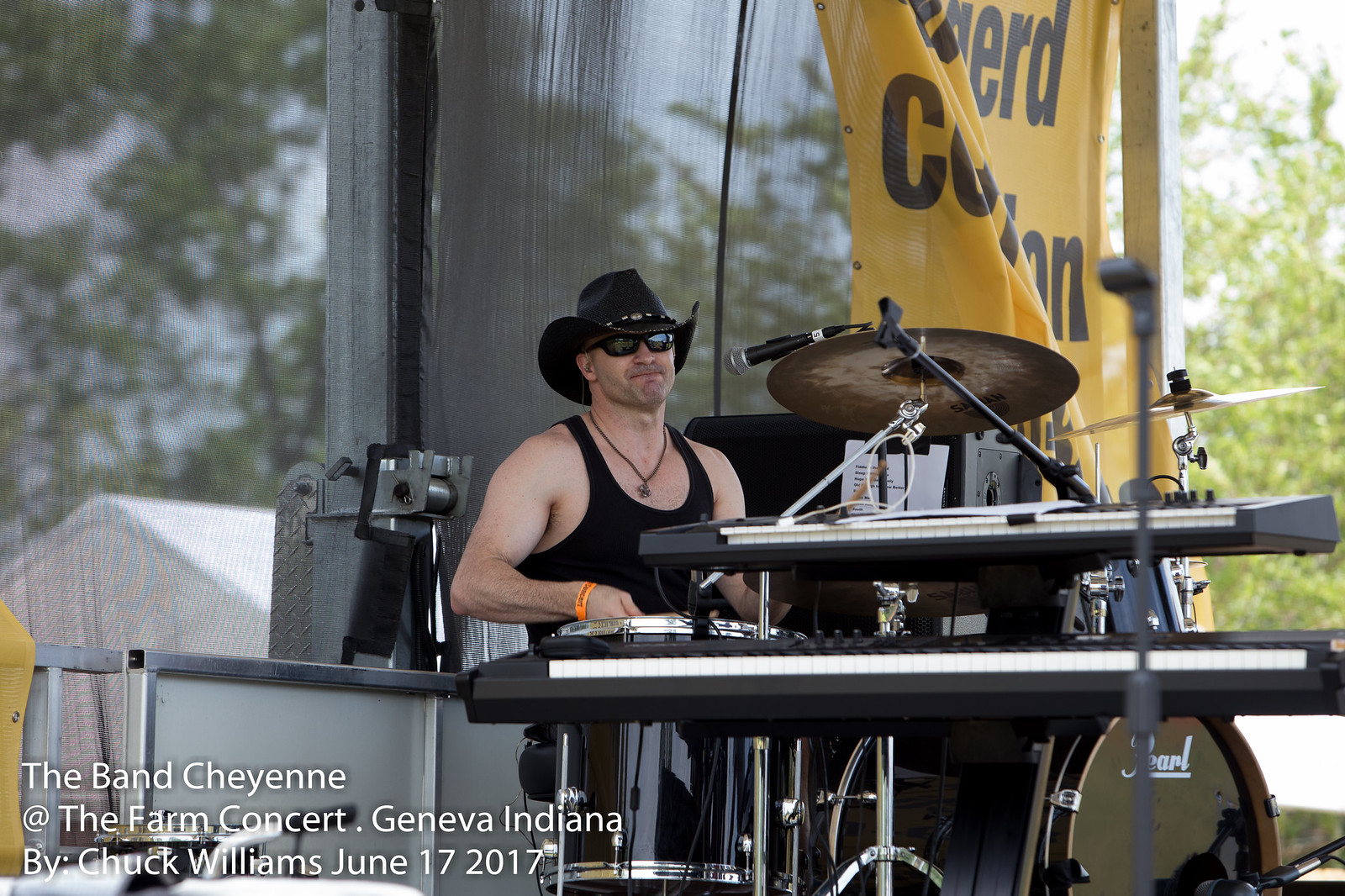This detailed picture captures a scene from the Farm Concert in Geneva, Indiana, featuring the band Cheyenne, as noted in white text in the lower left corner: "The band Cheyenne, the Farm Concert, Geneva, Indiana, by Chuck Williams, June 17, 2017." At the center of the image, a white male musician, likely in his 30s, is seen getting ready to play or performing. He is wearing a black sleeveless tank top, a cowboy hat, and dark sunglasses, with a necklace around his neck. He sits on a drum stool behind a Pearl drum kit, which includes a snare, bass drum, and two hi-hats. Positioned to his left is a microphone, indicating he might also be a vocalist. In front of him, just visible, is a two-level keyboard, suggesting proximity to the keyboardist. A semi-transparent screen behind him partially obscures the view of trees, a white shed or tent, enhancing the outdoor setting. A yellow banner with black text is also seen behind the drummer, though its inscription is difficult to read. The scene, devoid of other visible band members or much motion in the drummer's hands, suggests it might be captured just before the performance begins.